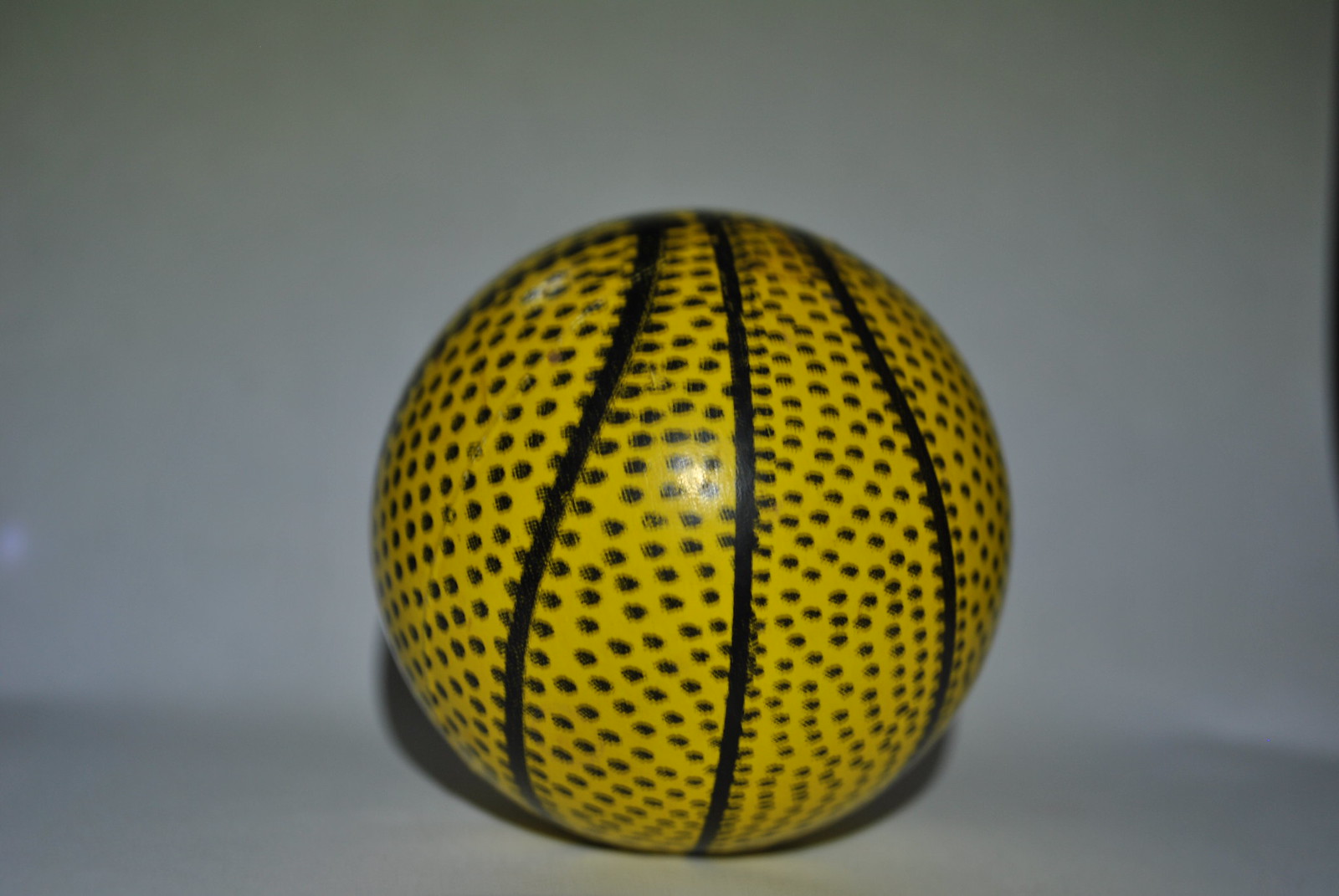The image showcases a detailed, close-up view of a yellow glass sculpture resembling a ball. The primary color is a vivid yellow, adorned with numerous small black dots that uniformly cover its surface, giving it a textured appearance. The ball features three distinct black stripes that vertically traverse the sphere, one running straight from top to bottom, flanked by two others that curve outward and come back toward the center. These lines create a pattern reminiscent of baseball or softball stitching but with an extra central stripe. The object is placed against a silver background, casting a slight shadow beneath it. A light source centered on the ball imparts a subtle, metallic shine. The overall intricate design and material suggest it is a piece of glass art, possibly a sculpture, rather than an actual sports ball.